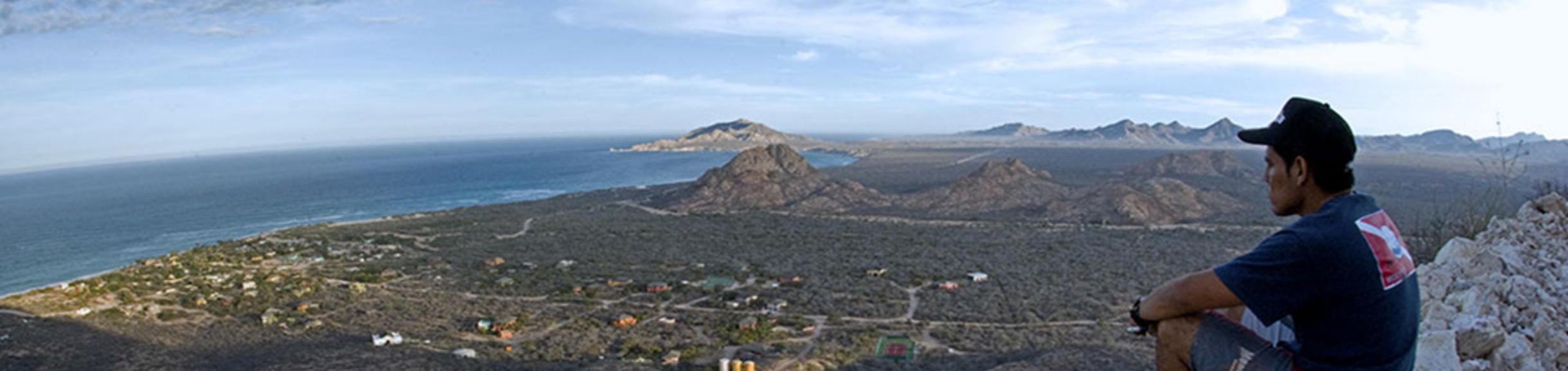The image depicts a young adult man, possibly of Mexican descent with tan skin, sitting on a white rocky formation. He is dressed in gray shorts, a navy blue t-shirt featuring a red rectangle with a white line through it on the back, and a dark-colored baseball cap. The man is positioned all the way to the right of the image, facing left, and appears to be taking in the panoramic view before him. The background reveals a vast, flat coastal landscape with a small city or town comprised of random streets and little houses extending towards a dark blue ocean. The scene is accentuated by big rocky mountains in the mid-ground and lighter brown rocky mountains in the far distance. The sky is blue with scattered white clouds, creating a serene backdrop to the man's contemplative pose, suggesting he might be on a hiking trip.